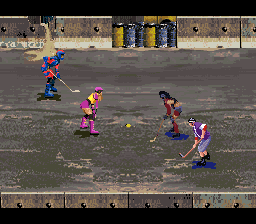This image is a screen capture from a retro-style video game, likely from the 16-bit or 64-bit era, featuring a street hockey match. The top 5-10% and bottom 5-10% of the image are bordered by black bars with cement breeze block walls, framing the playing area. In the center, four characters are positioned around a yellow ball, with two on the left and two on the right, each holding a hockey stick. The character in the lower right is a boy wearing a purple shirt and blue shorts, while above him stands a girl with long black hair, dressed in skimpy brown and denim attire. Opposite her is another girl in pink shorts, pink socks, boots, a yellow top, and a pink helmet. The final character in the upper left wears an orange and blue outfit. The overall color scheme is largely grey, accented by brightly colored characters. Along the top border, there are six large plastic drums - two yellow-green and four blue - contributing to the urban environment of the game.